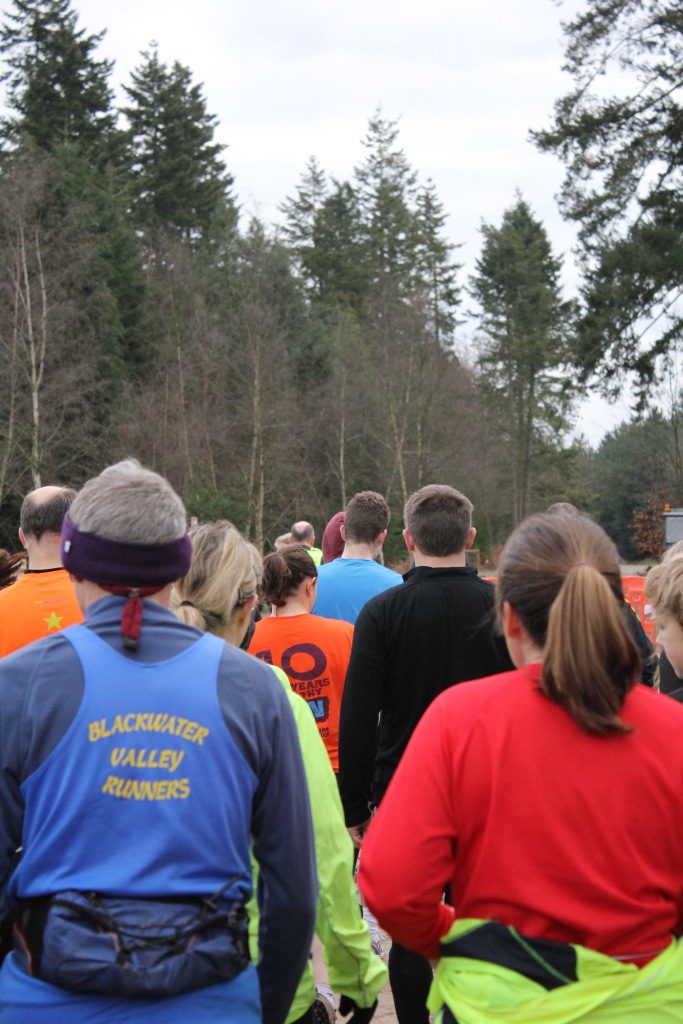The image depicts a vibrant and energetic scene in a wooded area, where a group of people, dressed in bright clothes—ranging from red to blue to orange to black—are gathered on a path, their backs facing the camera. The individuals appear to be preparing for an event, possibly a foot race or a hike, indicated by the natural setting and the mix of casual and athletic attire. Prominently featured, one man on the lower left wears a sleeveless T-shirt emblazoned with "Blackwater Rally Runners" and a headband, suggesting some participants might be part of a running group. The women, many with their hair pulled back, add to the impression of an imminent activity. Despite the presence of cloudy, gray skies above the towering trees, the photo is bright and clear, capturing the natural light of the outdoors. The image conveys a sense of anticipation and togetherness as the group faces a road ahead, ready for the journey that awaits.